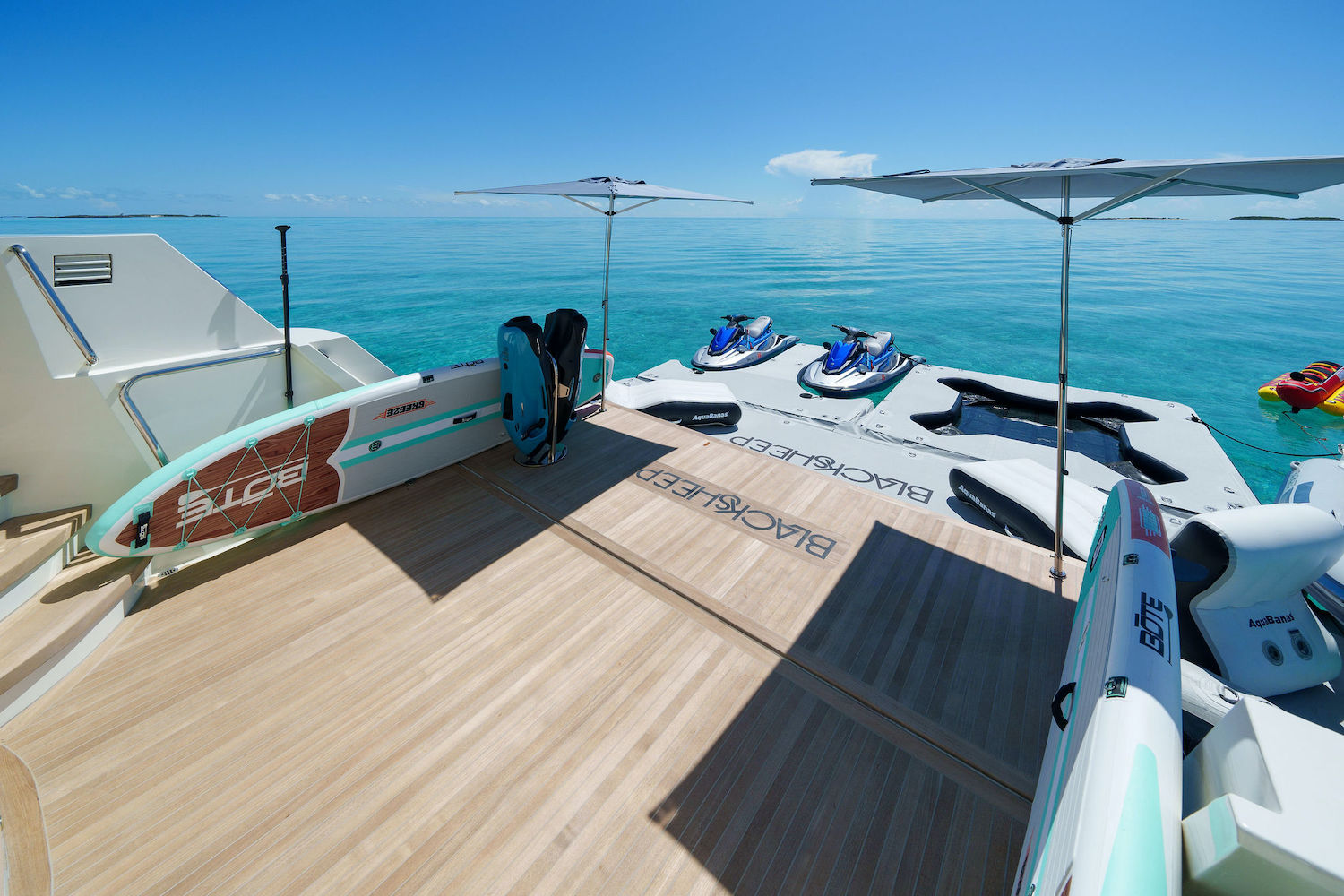The photograph captures the back deck of a boat, likely a yacht, designed for recreational use. The deck is composed of light brown wooden planks, which provide a warm and inviting surface. Centered prominently in the scene, two blue-gray umbrellas extend up from the wooden deck, offering a shaded respite from the sun. The deck's edge, marked by white railings, frames the sides of the image.

Towards the back of the boat, extending into the clear, turquoise blue water, there's an inflatable floating dock area. This additional structure features a small pool and several blow-up lounge chairs, enhancing the boat's leisure amenities. Attached to this floating dock are two sleek jet skis, painted in blue and gray hues, ready for exhilarating rides across the serene waters.

The pristine clarity of the water allows one to see the seabed, emphasizing the tropical, crystal-clear environment. In the distance, the horizon is marked by a barely visible thin line of clouds, under an expansive bright blue sky. The phrase "Black Sheep" is emblazoned on both the wooden deck of the boat and the attached floating dock area, tying the scene together with a sense of identity and branding.